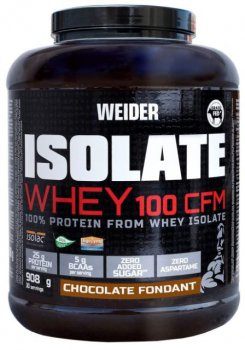This product photography image showcases a premium canister of protein powder, ideal for fitness enthusiasts and gym-goers. The packaging is a sleek black plastic container, prominently featuring the brand's name and product details in bold, eye-catching text. At the top, in smaller white letters, is the brand name "WIDER." Just below it, "ISOLATE" is displayed in large, white block letters, ensuring immediate recognition. Below this, the designation "WHEY 100-C-F-M" appears in striking red text. Accompanying these details, the phrase "100% Protein from WHEY ISOLATE" is also visible in white text, emphasizing the product's purity and protein content. Further down, there are organized boxes highlighting nutritional details such as sugar and protein content. Finally, at the very bottom, the flavor is specified in a brown box labeled "CHOCOLATE FONDANT."